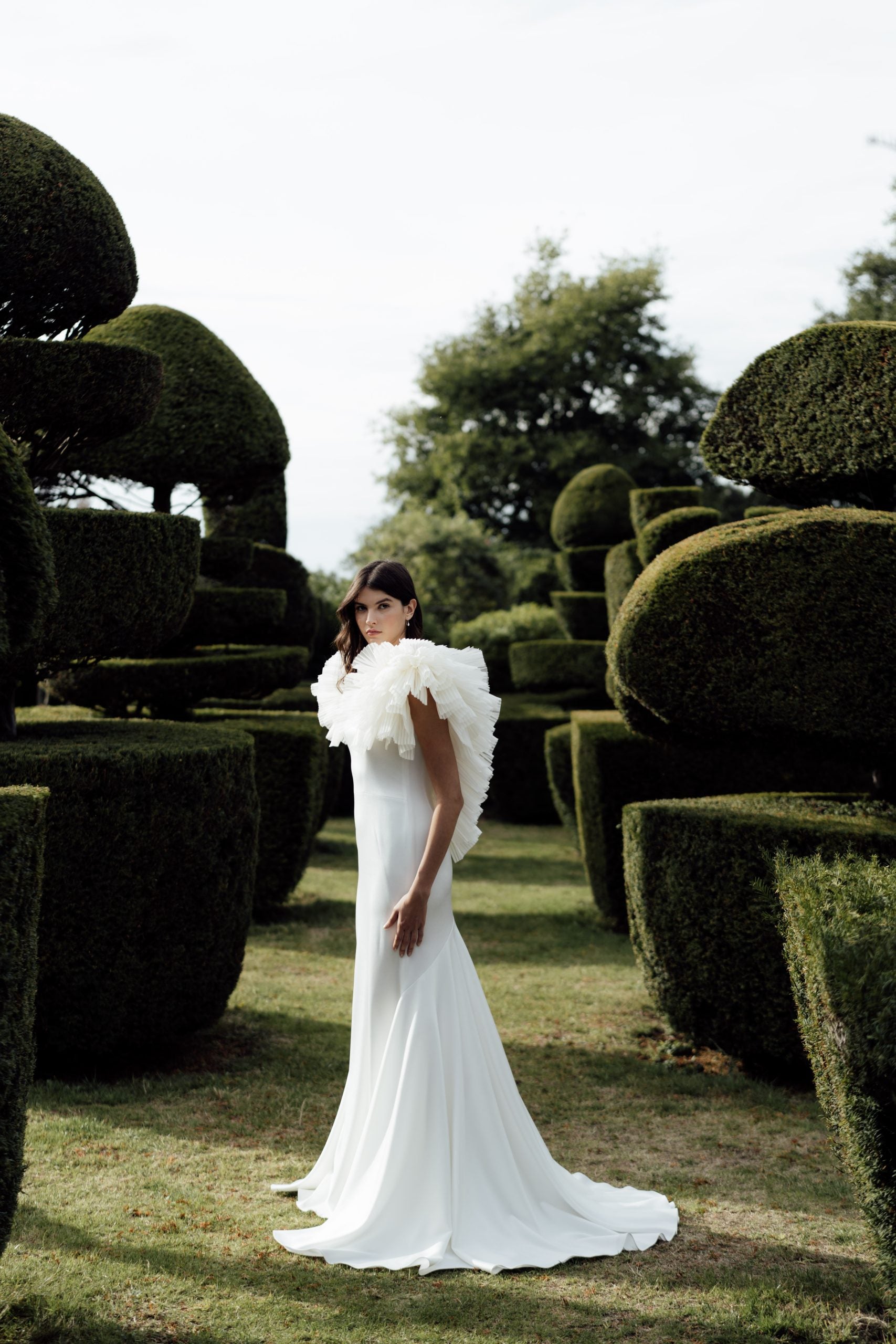In a meticulously manicured garden featuring well-trimmed bushes and abstract topiaries, a tall, beautiful fashion model stands elegantly in profile, her head turned toward the camera. She has striking dark hair, fair skin, and red lips. Dressed in a sleek, long white gown reminiscent of a wedding dress, the fabric fits her frame closely before flaring out and spreading across the lush green grass. The dress features short sleeves and an elaborate ruffled collar that extends from around her neck, cascading down her back to her lower back. Standing amidst the sculpted greenery, her arm relaxed at her side, she captures a sense of serene poise and grace while gazing directly at the camera.